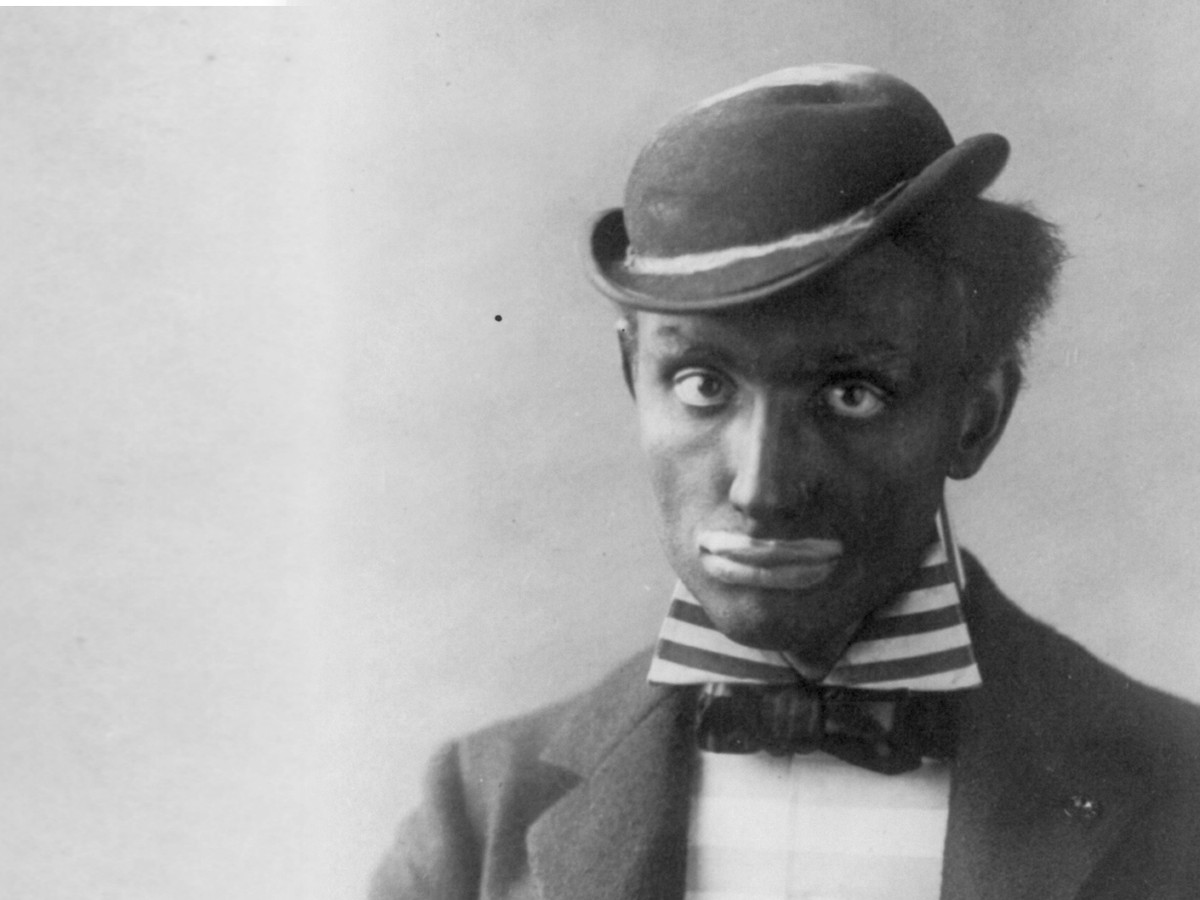In this early 20th-century black-and-white photograph, a man, possibly a performer or mime, is portrayed with striking details. The man appears to be in blackface, with dark makeup covering his face and his lips prominently painted, which resemble the use of heavy lipstick or lip gloss. His expression is one of surprise, with wide eyes staring directly at the camera. He wears a small, slightly tilted bowler hat that has a short rim and is styled with a bowl shape on top. His attire consists of a dark suit jacket, likely wool, over a white shirt with a striped collar and a small black bow tie. There seems to be a hint of a scarf or additional fabric beneath his collar. The background is a plain gray wall, providing a stark contrast to his detailed and expressive appearance. His hair is short and slightly sticking out from the sides of the hat. The overall composition and the man’s evocative attire suggest he is likely a performer attempting to convey a mimetic or clownish character.